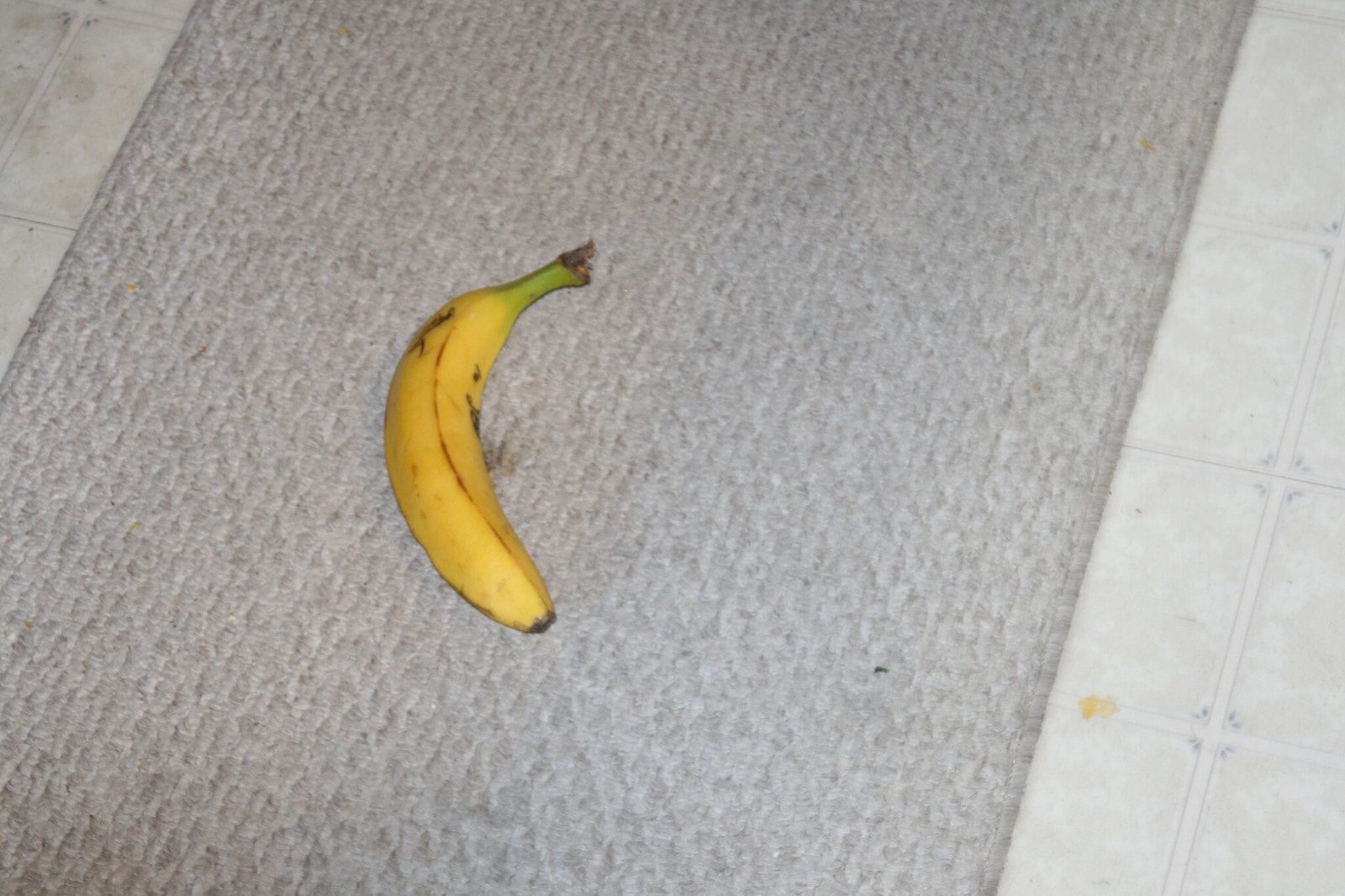A light gray tile floor is shown, featuring a small reddish-yellow spot near the bottom right corner. Centered in the image is a light gray rug, upon which a ripe banana rests. The banana is predominantly yellow with a green stem and dark spots scattered across its peel. It has a notable brown line running down its length, complemented by a small black spot in the center and a few additional bruises. The banana is slightly plump and not too long. In the upper left corner of the image, there are small dark marks on the floor that resemble grease or spilled drink stains. Despite the bruises, the banana appears fresh and appetizing.